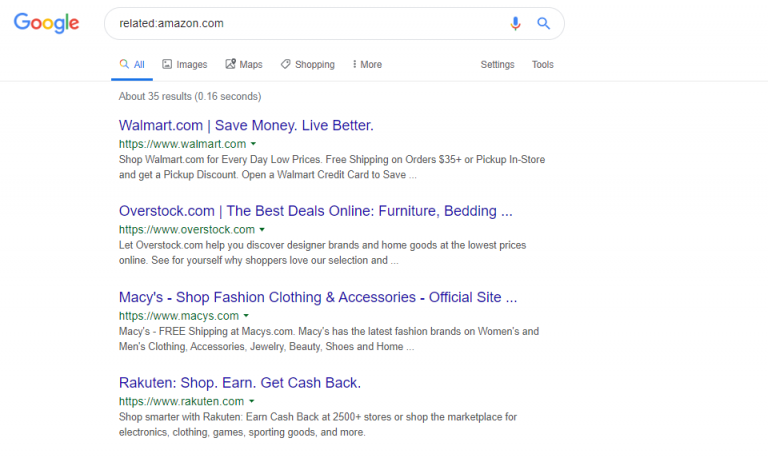The image displays a Google search results page with the classic Google logo in the upper left corner, consisting of the letters 'G', 'o', 'o', 'g', 'l', and 'e' in blue, red, yellow, blue, green, and red respectively. The webpage features a clean, white background. The search term entered into the search box is "related:amazon.com," a query designed to find websites similar to Amazon.

Below the search bar, under the "All" tab, the screenshot shows four search results out of a total of approximately 35. The first result is Walmart's official website (walmart.com) with the tagline "Save Money, Look Better." The second result is Overstock (overstock.com), promising "the best deals online" for furniture and bedding. The third result is Macy's official site (macys.com), marketing itself with "Shop Fashion, Clothing and Accessories." The final result visible in the screenshot is Rakuten (rakuten.com), which highlights "Shop, Earn, Get Cash Back."

Each link includes a brief description emphasizing that these websites are primarily shopping platforms offering various products such as clothing, goods, groceries, and other items.